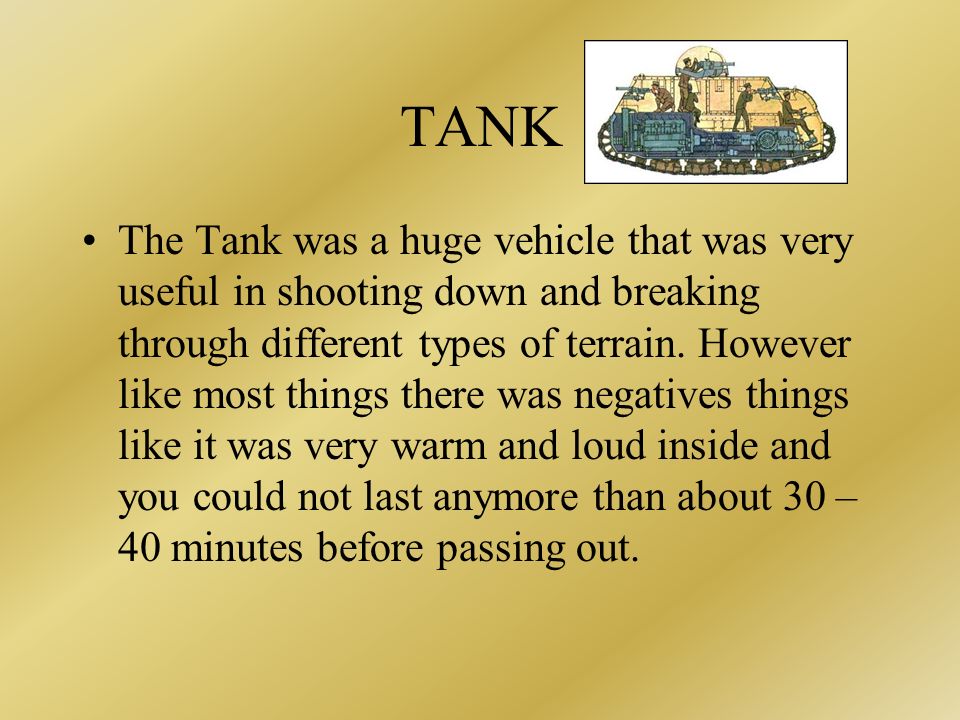The rectangular image features a detailed, variegated yellowy-gold background. Prominently in the upper right, an illustrated diagram of a tank reveals its interior, showing soldiers in various positions: one at the front, two firing from the front and back, and another manning a machine gun in the turret. To the left of this illustration, the word "TANK" is displayed in solid black, uppercase letters. Beneath, a bullet point in smaller black font explains: "The tank was a huge vehicle that was very useful in shooting down and breaking through different types of terrain. However, like most things, there were negatives. It was very warm and loud inside, and you could not last more than about 30 to 40 minutes before passing out."